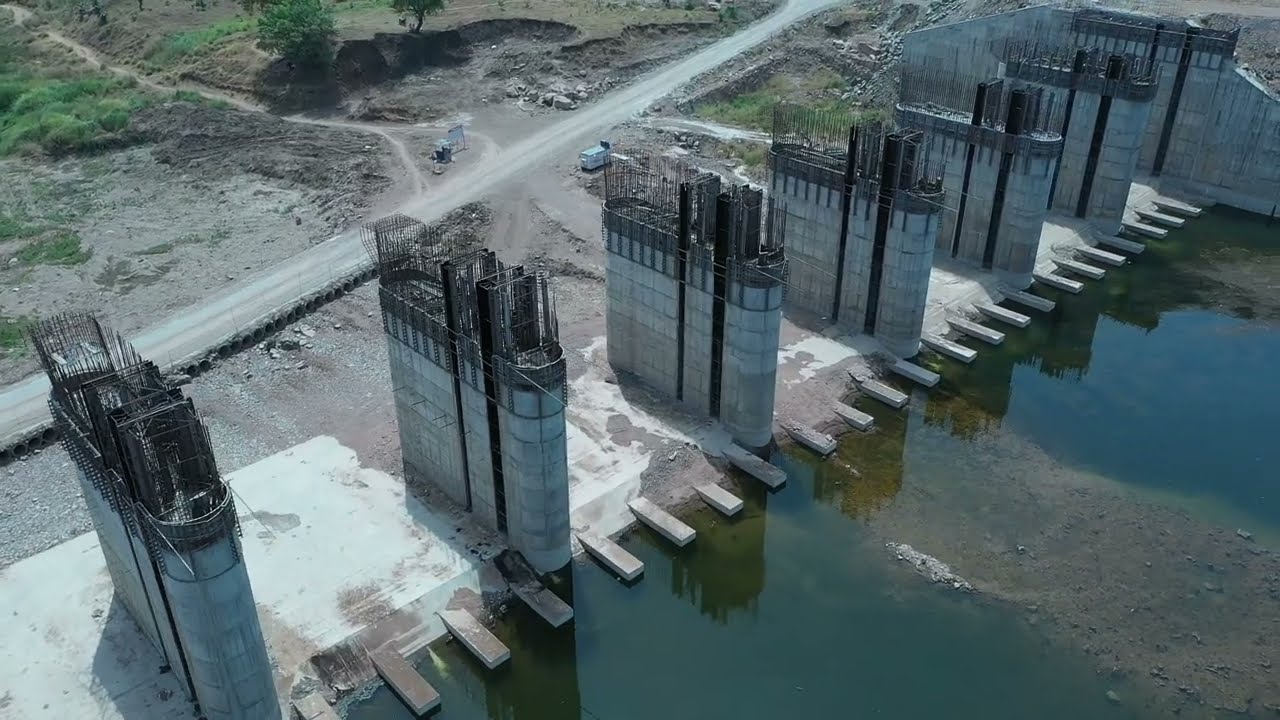The image depicts an early-stage construction site at a waterway that appears to be the foundation for a bridge or a similar structure. The central feature is a series of six large, off-white concrete pillars aligned diagonally from the bottom left to the top right of the image. These pillars are situated on a cement platform, each topped with protruding metal rods, indicating ongoing construction. Along the platform, near the bottom right, are metal structures resembling the teeth of a comb.

To the lower right of the image, a waterway with visible dirt and rock sediment runs centrally, and the water itself is shallow. The right side of the cement slab has small, wood-like protrusions. In the background, there is a road or pathway running parallel to the construction site from the middle left to the top middle of the image, behind which erosion and ongoing construction activities are evident. Sparse vegetation, including small shrubs and a tree or bush, is visible at the upper left of the image.